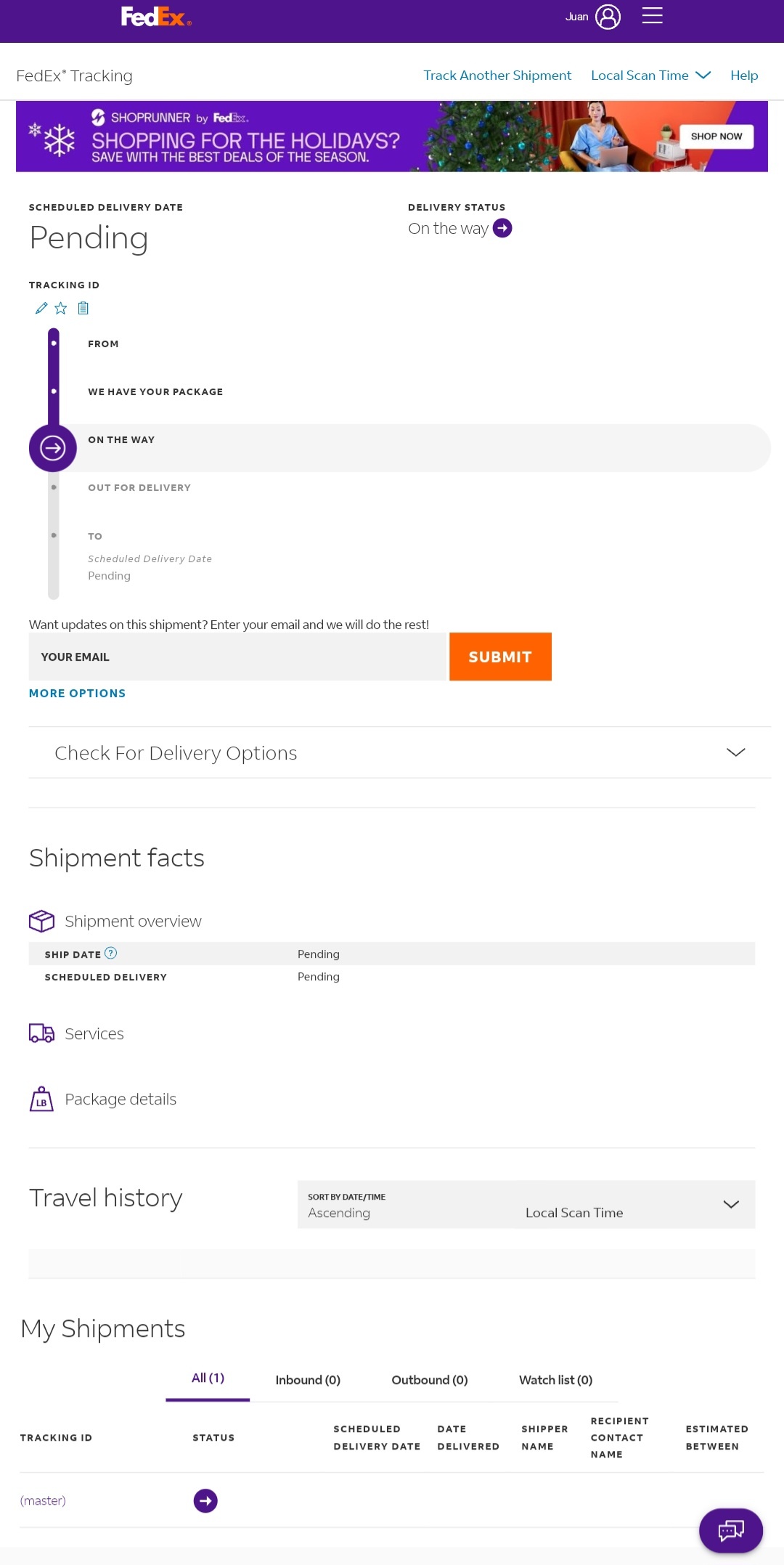The image depicts a scene from the FedEx website. At the top, there is a prominent purple navigation bar. On the right side of this bar, “FedEx” is displayed in their iconic style, with "Fed" in white and "Ex" in red. The "F" and the "E" are capitalized, while the other letters are in lowercase.

Below this bar, there is a white section that includes a variety of options. It features "FedEx Tracking" on the left, and on the right, options for "Track Another Shipment," "Local Scan Time," and "Help."

Another purple bar follows, containing a holiday-themed message in white text: "Shopping for the holidays, save with the best deals of the season." Above this bar on the left, there is an image of a snowflake, and on the right, there are visuals of a Christmas tree and a woman sitting in a chair with a laptop. The backdrop features an orange wall, and a white button labeled "Shop Now" is prominently displayed.

Below this, on the left side, there are delivery status updates with "Schedule Delivery Date Pending" and "Delivery Status On the Way." Under the "Pending" section, it specifies the tracking ID and further details with phrases like "We have your package," "On the way," and "Out for delivery." There's also a box provided for users to submit their email.

Following these sections, there are additional options for "Check for Delivery Options," "Shipment Facts," "Shipment Overview," "Services," "Package Deals," "Travel History," and "My Shipments," where users can manage their shipments. In the lower left corner, there is a purple button available for speaking with a customer service representative for assistance.